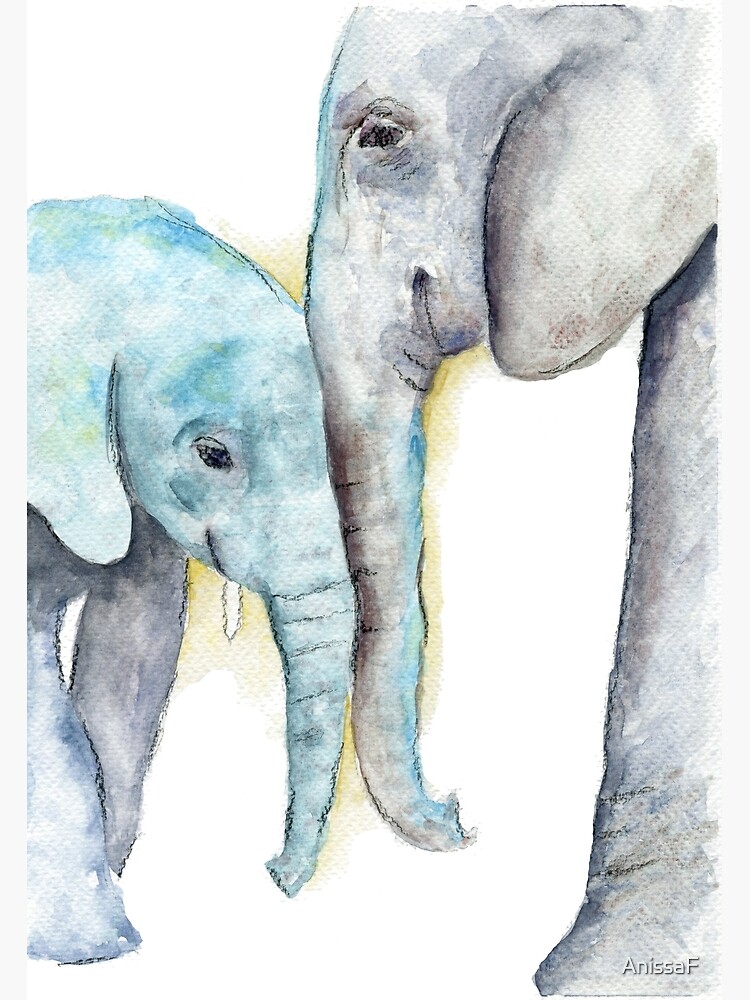This is a watercolor painting created by artist Anissa F, as indicated by the copyright or watermark in the bottom right corner. It depicts a touching scene between two elephants – an adult on the right and a younger one on the left. The adult elephant, which could be either a mother or father, is standing tall, occupying the length of the portrait from top to bottom. It is primarily gray, with its head pointed downwards as its trunk delicately touches the face of the child elephant. 

The young elephant, positioned to the left and facing the adult, has a bluish hue around its head, ears, and trunk, with its legs appearing more gray. The baby elephant also has a small visible tusk. Their trunks are entwined in an endearing manner that resembles an "elephant-style hug." Surrounding their trunks are subtle yellowish-green markings that add depth and a background element to the composition. This detailed and tender portrayal highlights the bond between the elephants, making it a lovely and heartwarming piece.